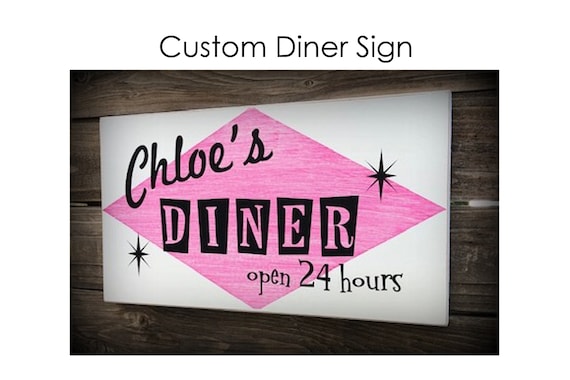The image is an advertisement for a custom diner sign. It features a photograph of a framed white rectangular sign set against a dark brown, wooden wall. The sign is wider on the right side than the left, adding an irregular, angled dimension to its appearance. In the center of the sign is a bright, pink diamond shape oriented from top left to bottom right. Overlaid on the diamond shape, the name "Chloe's" is written in bold, cursive black letters. Below that, the word "Diner" is displayed in a unique style where each letter is pink with a distinct black square background, giving a cut-out effect. Beneath "Diner," the text "Open 24 Hours" is printed in straightforward black letters. Adding decorative detail, there are two black stars—one slightly above and to the right of the "R" in "Diner," and another to the left below the "D."